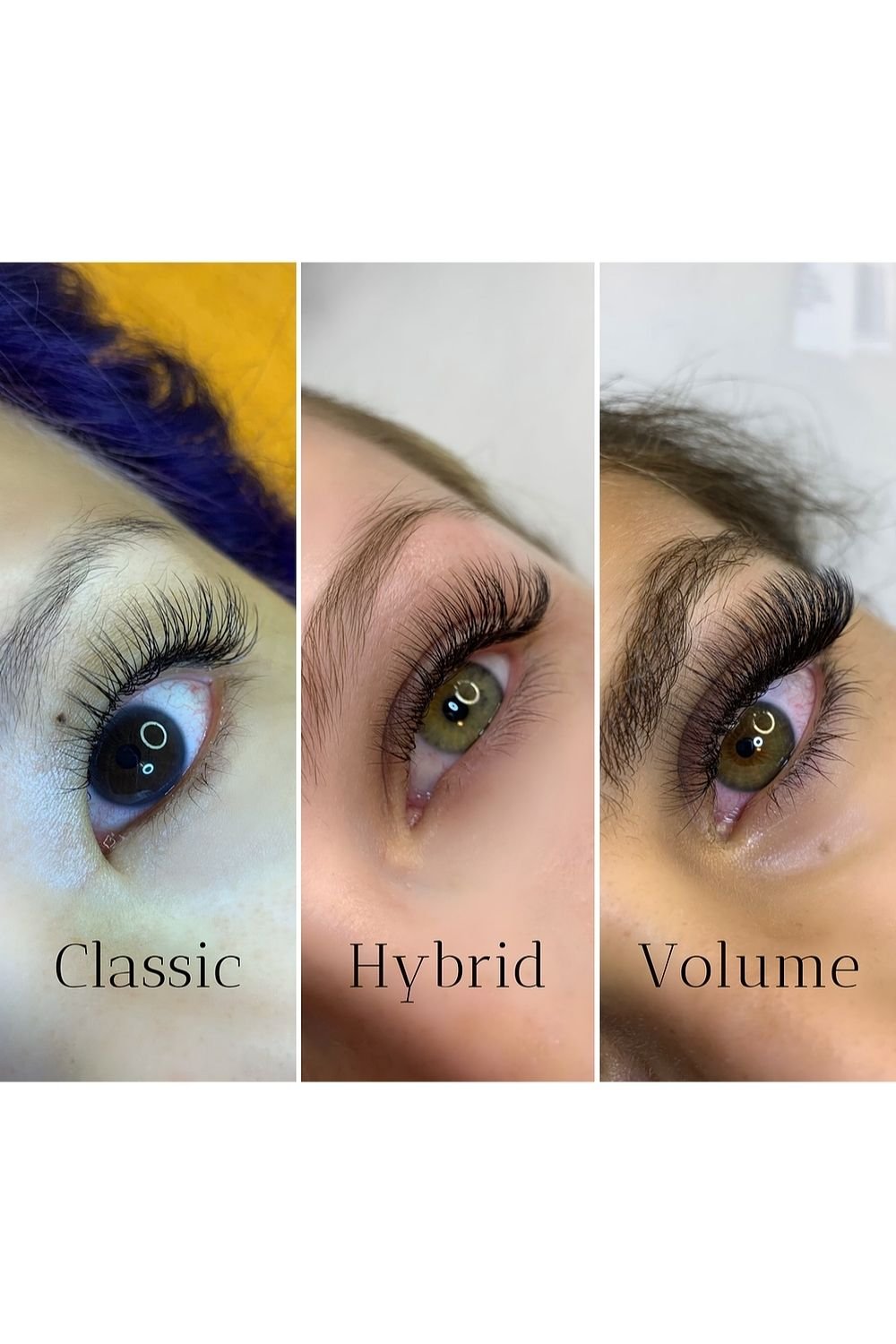The image consists of three vertically aligned, side-by-side close-up pictures of a woman's eye and part of her face, each heavily filtered to highlight different aspects of her appearance. Each filter is labeled: the first picture is labeled "Classic," the second "Hybrid," and the third "Volume."

In the "Classic" picture, the woman's skin has a greenish tint, with her eye appearing completely black. Her hair is blue, and the background is yellow, with a notable greenish spot where her highlight is. 

The "Hybrid" picture shows her with a more natural appearance: she has green eyes, brownish hair, and dark eyelashes. Her skin tone is normal, and only a little bit of her brown hair is visible. The background appears white.

In the "Volume" picture, the woman has coarse black eyebrows and fuzzy black hair, with her greenish eye standing out prominently. Her eyelashes appear significantly thicker, and her skin tone remains normal.

The images collectively illustrate varying appearances of the same woman using different camera filters, enhancing different facial features and colors in each version.